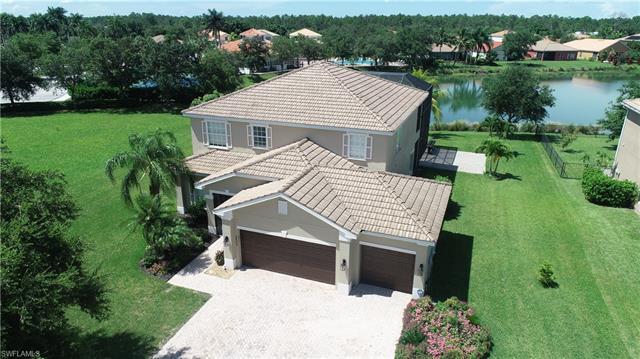This is an aerial view of a two-story, Spanish-style single-family home located in a residential community in Florida. The house features a three-car garage with tan and brown doors, where the door on the left is wider than the one on the right. The exterior is cream-colored stucco with tile roofing. Palm trees grace the entryway near the front door, enhancing the lush appearance of the green grass that covers the large yards surrounding the home. The spacious backyard, which includes a fenced and covered pool, extends to a man-made lake or pond, adding to the serene setting. Neighboring homes are visible around the property, contributing to the community feel.